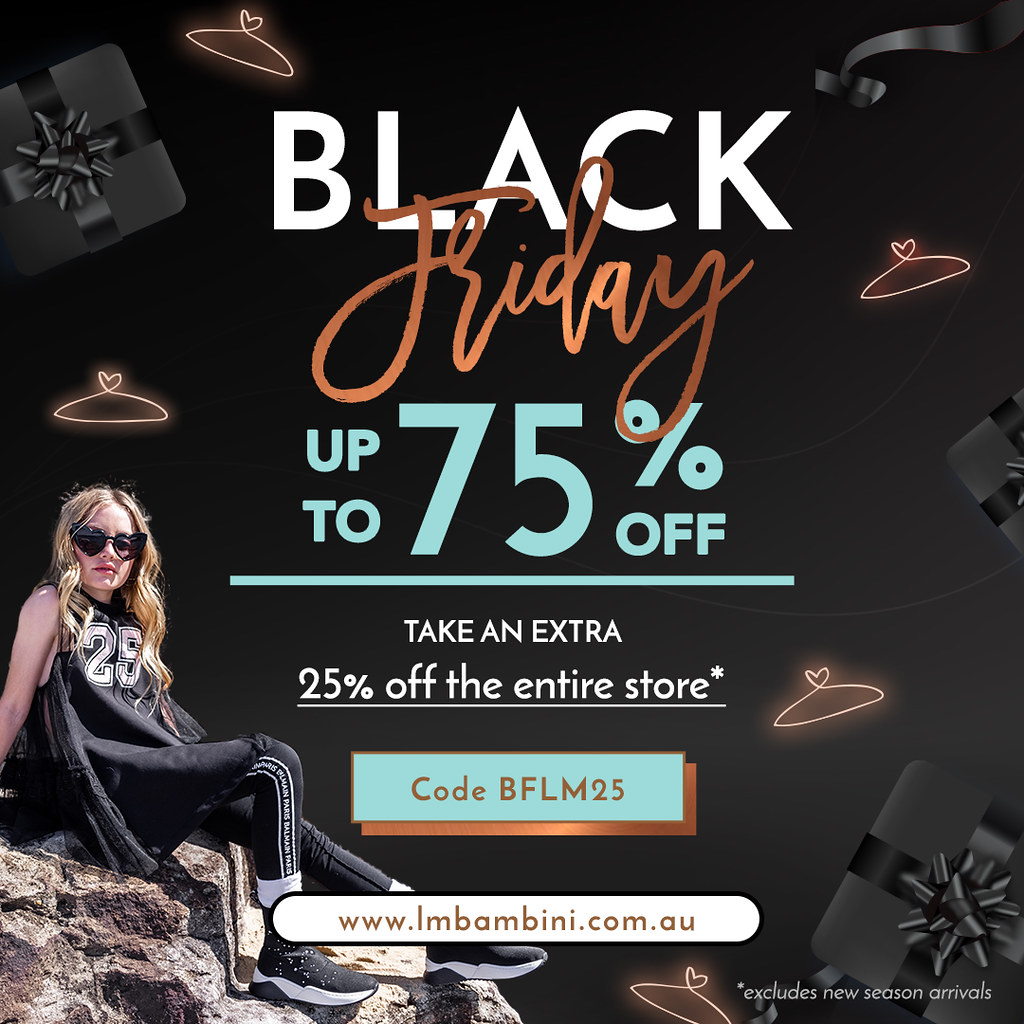The advertisement features a sleek, modern design set against a black background, with various elements strategically placed to catch the eye. Floating around in the background are stylish, black-wrapped presents with black ribbons and unique neon coat hangers that have hearts instead of hooks. On the left side, a young woman, possibly in her early 20s, is prominently photoshopped sitting on a rock. She is decked out in a black jersey, black spandex pants, black tennis shoes, and black sunglasses, her blonde hair adding a touch of contrast.

At the center of the image is the main promotional text: "Black Friday up to 75% off," with "Friday" in a cursive script that mimics gold, "Black" in white, and "up to 75%" in blue. Below that, it mentions an additional offer: "take an extra 25% off the entire store," followed by a call-to-action button in blue and gold providing a discount code, "BFLM25." Along the bottom, there’s an oval button displaying the website address, "lmbini.com.au". The advertisement makes it clear that new season arrivals are excluded from the sale. 

Overall, the design is visually striking and packed with information, making it a comprehensive and enticing Black Friday promotion.